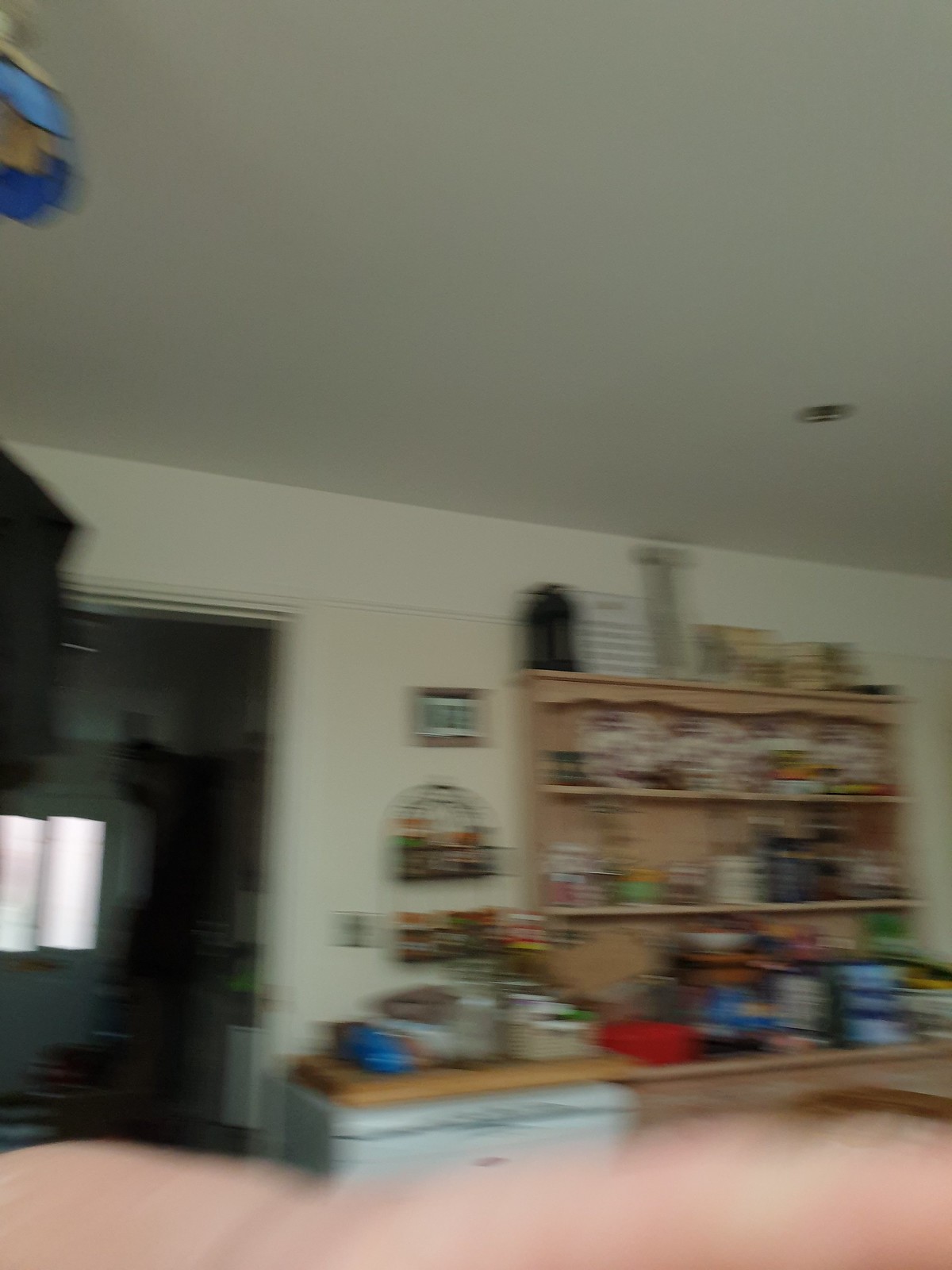In this slightly blurry photograph of a kitchen area, the foreground is partially obscured by a pinkish hue, likely from a finger caught in the frame. The kitchen features a white ceiling and matching back walls. A doorway opens into a darker adjacent room filled with items in brown, gray, and black tones. Prominently featured in the kitchen is a tan, three-tiered shelving unit. The top shelf is adorned with various decor pieces, while the second shelf holds white and purple plates. The bottom two shelves are stocked with an assortment of cans and canisters. Additionally, a white cabinet with a light brown butcher block top is visible, holding more containers and adding to the kitchen storage options.